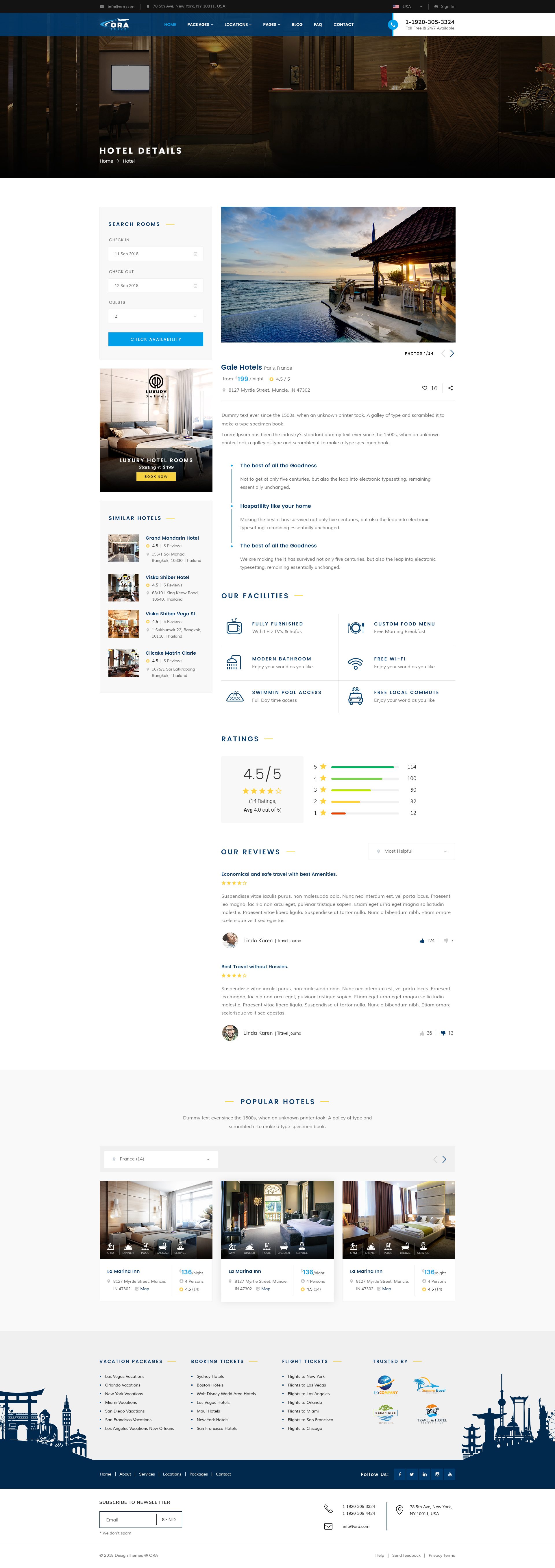**Caption:**

This screenshot captures a heavily consolidated image of a large website, primarily featuring hotel information. 

- **Header Area:** At the top, a dark brown banner spans the width of the page, depicting a snippet of furniture and a wall-mounted light fixture. To the left, a blue bar runs horizontally, showcasing bold white lettering that appears to spell "OBA" or "OSA." Adjacent to this, a series of white labels extends rightwards, culminating in a white rectangle in the upper right corner, seemingly containing a phone number. The bottom left corner of the dark brown section reads "Hotel Details" in white text against the brown background.

- **Main Content Section:** Below the brown banner, the background turns white. The left side is layered with various words and labels, while the right side prominently features an image suggesting a Tahitian or Bali-style resort overlooking the water at sunset. There is also a distinct blue rectangular bar on the left side, beneath which sits a square image. A logo on a white wall appears to have been taken from inside a hotel room, with the phrase "luxury hotel rooms" discernible in white text at the bottom of the image.

- **Additional Elements:** Below this, the text "similar hotels" appears on a white background. A column of four small images lines the left side, flanking blue headers and a hotel name that is too small to read. Centrally located, beneath the primary resort image, the text "Gale Hotels" is displayed in blue, followed by an array of black wording. The page is divided into three sections, each demarcated by dark blue text, though specifics are indistinguishable.

- **Details and Ratings:** Visible below, the phrase "our facilities" is printed in larger text, alongside a series of tiny blue icons. A rating bar reveals a score of 4.5 out of 5 stars on the left side, whereas the right presents a bar chart, depicting ratings from 1 to 5 with green, yellow, and red bars.

- **Reviews and Footer:** The section titled "Reviews" in bold blue letters includes a few paragraphs of information, complete with blue headlines and user icons, though specifics remain indistinct due to the reduction. The page concludes with a gray footer labeled "Popular Hotels" in small text, and showcases three images of hotel rooms, each with identifying blue headlines beneath. The bottom-most portion features a white background trimmed with a black banner, displaying silhouettes of Asian motifs like Buddha and pagodas on the left. These thematic designs extend to the right, incorporating Arab and South American artifacts in a similar silhouette style.

Overall, the intricate layout hints at the website's focus on hotel details, amenities, and user reviews, accentuated by culturally rich visuals.